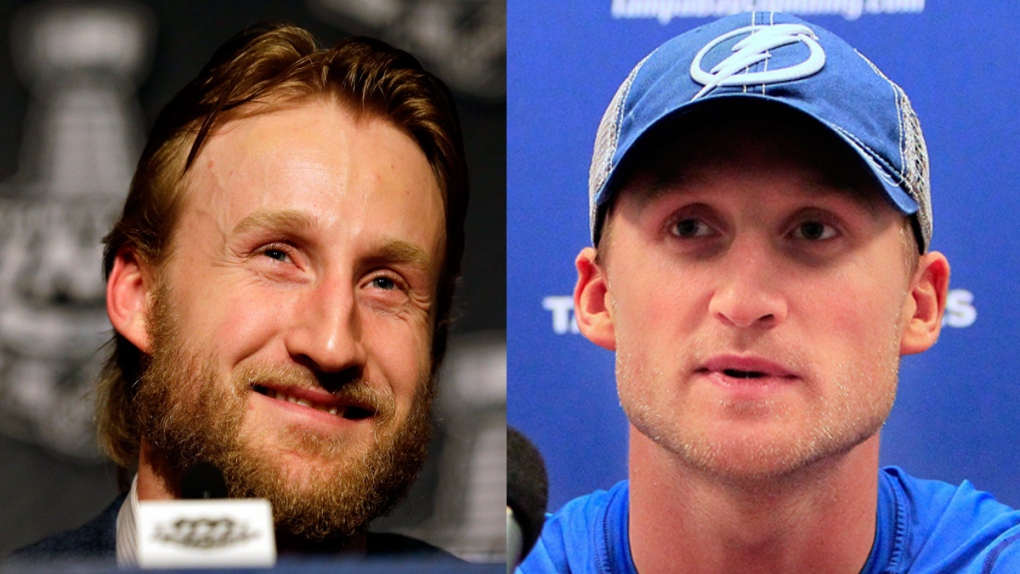The image features two men positioned side by side in separate squares with a blurred background. In the left square, there's a white male with a big forehead and brown, mid-length hair that's slicked back. He sports a dark brown beard and has a distinctive smile. A possible microphone is visible in the foreground, suggesting he might be in an interview setting. The man on the left also has a name tag beneath him. 

On the right side, a white male is seen wearing a blue baseball cap with a lightning logo and a blue shirt. This man has a closely-trimmed stubble and appears to be speaking, as indicated by his open mouth and focused gaze into the distance. The background behind him is predominantly blue with text that is mostly unreadable due to obstruction. Another microphone is also present in this part of the image, reinforcing the interview scenario.